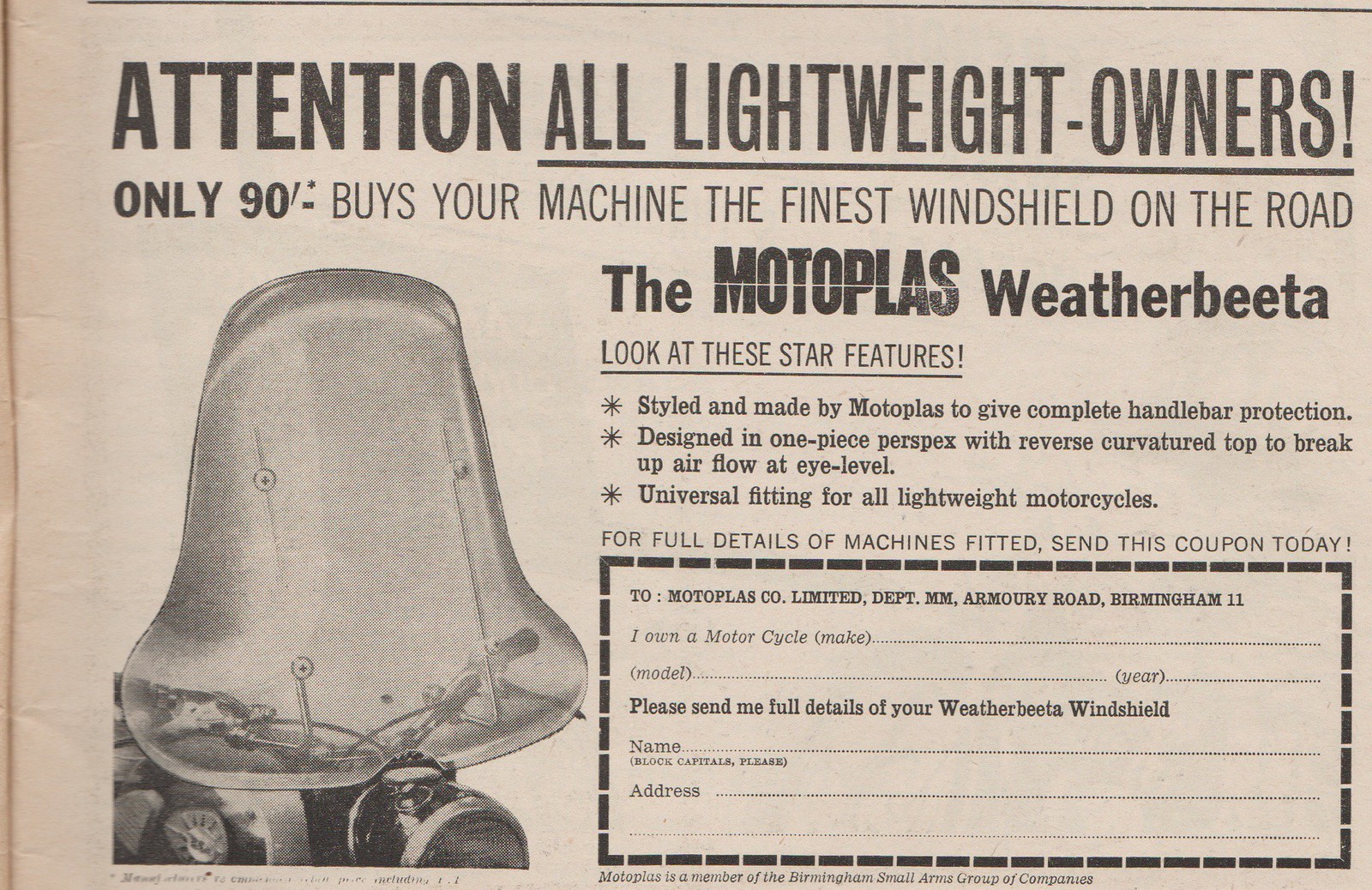Certainly! Here is a consolidated and detailed caption incorporating the details from each contribution:

---

The image depicts an advertisement, likely from the middle of a vintage magazine or possibly an old, faded newspaper. The top of the ad shouts in bold letters: "Attention all lightweight owners! Only $90 buys your machine the finest windshield on the road." It introduces the product as the "Motoplace Weather Beta," and features a prominent image of a motorcycle windshield on the left side. The ad highlights the key benefits with star features:

- Styled and made by Motoplace for complete handlebar protection.
- Designed in one piece per specs with a reverse curvature top to break up airflow at eye level.
- Universal fitting suitable for all lightweight motorcycles.

Below these bullet points, there's a coupon section, delineated by a dotted line, where prospective buyers can provide details about their motorcycle (make, model, and year) along with their personal information (name and address). The full details of machines fitted can be obtained by sending this filled-out coupon to Motoplace Limited, M.M. Armory Road, Birmingham 11. Additionally, the ad mentions that Motoplace is a member of the Birmingham Small Arms Group of Companies.